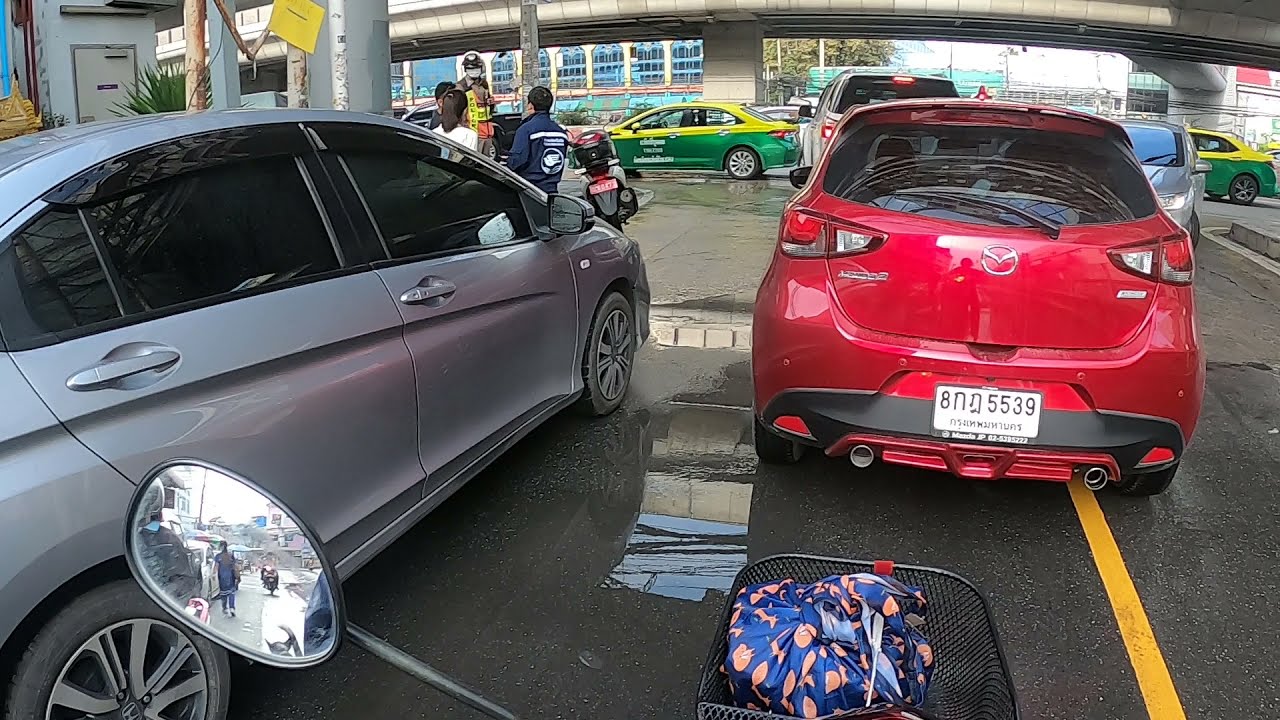The image depicts a busy parking lot scene, viewed from the perspective of someone on a motorbike or scooter. The foreground reveals the scooter's handlebar, a rearview mirror, and a basket containing a blue and orange bag. The parking lot surface appears wet, indicating recent rainfall and creating small puddles. Directly ahead, a red Mazda hatchback is visible, albeit in a chaotic setting where vehicles seem improperly parked or maneuvering haphazardly. A gray car with black-tinted windows is positioned to the left, while another vehicle is obstructing the path of the red car from the right. Further along, two green and yellow taxis are lined up, and barely visible behind the rider is another motorcycle. The background features additional cars, a bridge or pedestrian walkway, and some buildings. Near the gray car, a small group of people, possibly including a traffic officer, seem engaged in conversation, adding to the overall impression of a congested and disordered environment.